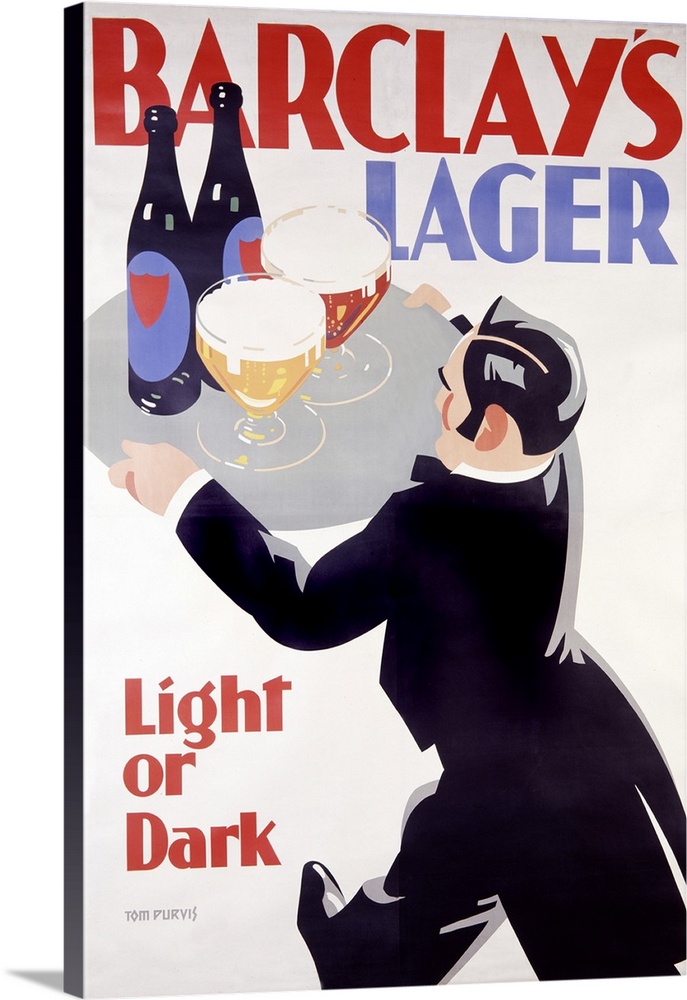The image appears to be a vintage-style book cover or advertisement featuring a cartoon illustration with a white background. At the top, the title "Barclays Lager" is prominently displayed, with "Barclays" in red and "Lager" in blue or purple depending on the description. A waiter or bartender, dressed in an old-fashioned black suit with coattails and polished black hair combed tightly back, is centrally depicted. 

This character is holding a large tray, which carries two tall purple or blue bottles and two large glasses—one a creamy color, the other a dark burgundy. In the bottom left corner, the text "light or dark" appears in red, with the word "light" being somewhat faded. Additionally, the name "Tom Purvis" is inscribed in small light gray text at the bottom left. The book or sign is angled slightly to the left, casting a slight shadow on that side.